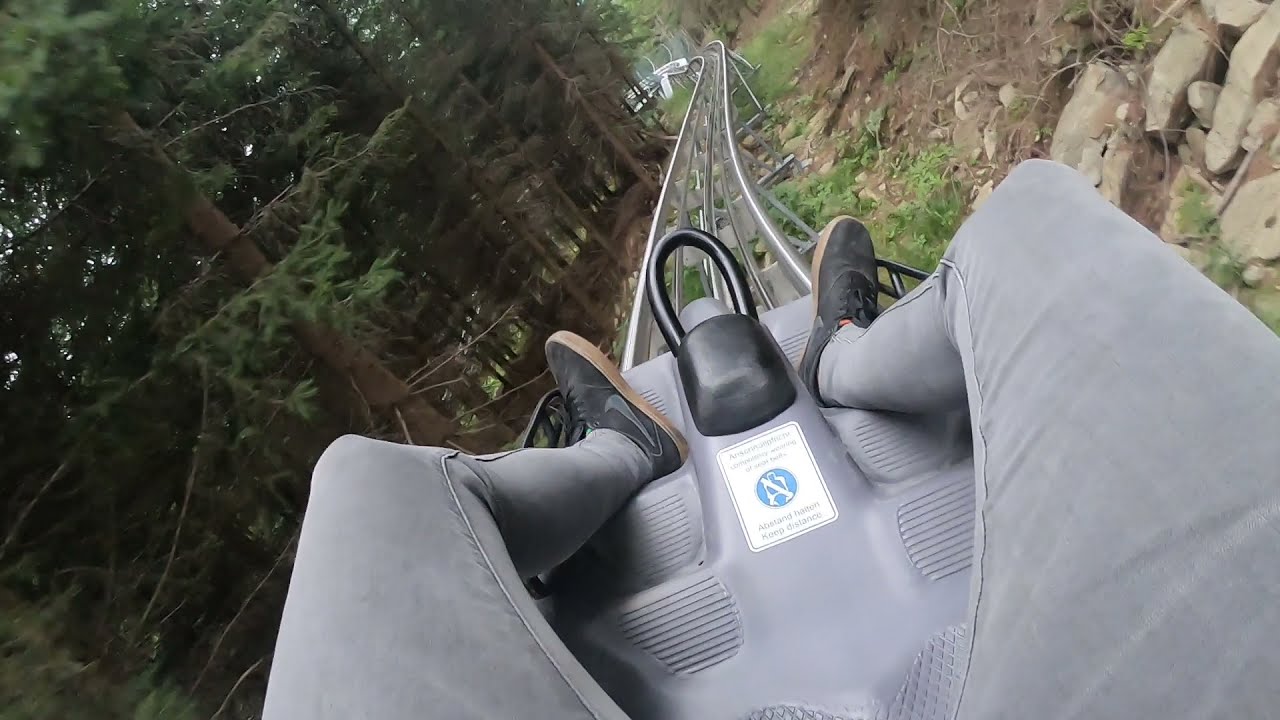The image is a wide rectangular daytime shot capturing a first-person view from a rider sitting on a roller coaster-like track ride. The rider's legs are in the bottom right corner, extending forward in gray, tight-fitting pants. The feet, clad in black Nike shoes with gray logos and gum soles, rest on a gray contraption likely made of metal. A white warning label with a blue logo is visible on the cart, and there's a black metal loop or hook in front. The track itself, metallic and unpainted, winds through a natural outdoor setting. On the left side of the track are numerous evergreen trees, hinting at a dense forest. To the right, there's a rocky hillside, where the land has been cleared to accommodate the track.